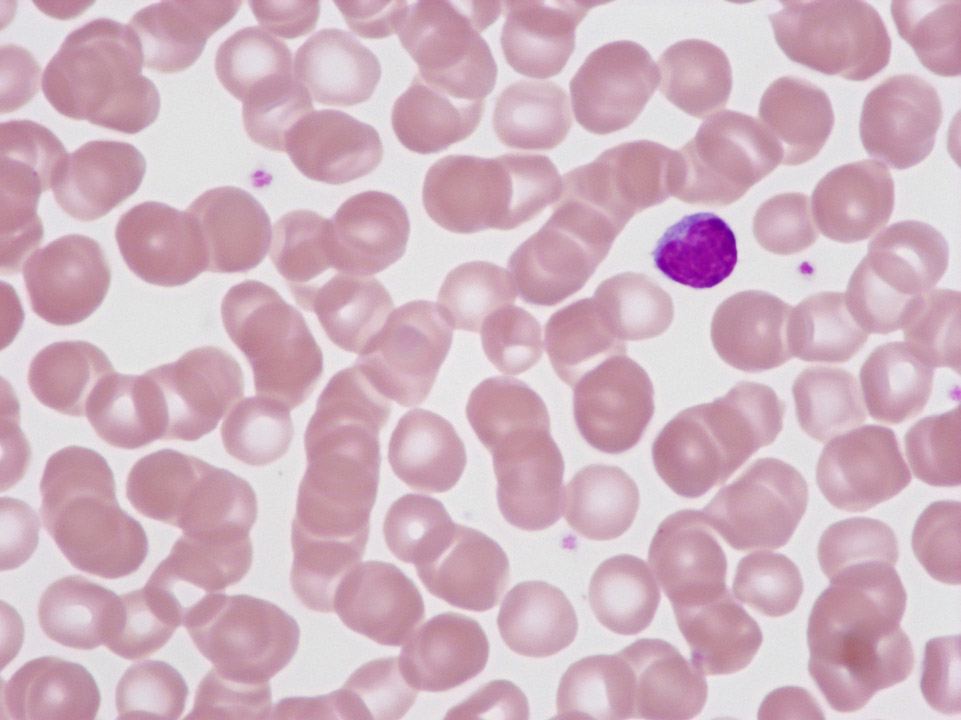This is a highly detailed microscopic image of cells, likely stained with dye to highlight specific structures. The image displays a square frame filled with numerous pink, round shapes scattered throughout. The cells form various patterns, including random lines, curlicues, and even a distinct U-shape. Notably, many of the cells appear semi-transparent with a lighter pink hue against a pristine white background. 

Concentrated towards the top-right quadrant, a prominent dark purple round blob stands out, accompanied by a much smaller dot nearby. On the opposite side, near the top-left corner, another tiny dot—resembling the size of a pencil-dot—is visible. The image appears to be specifically stained, potentially to identify significant markers such as cancer cells. Overall, this detailed view offers a fascinating insight into cellular structures and potential abnormalities.